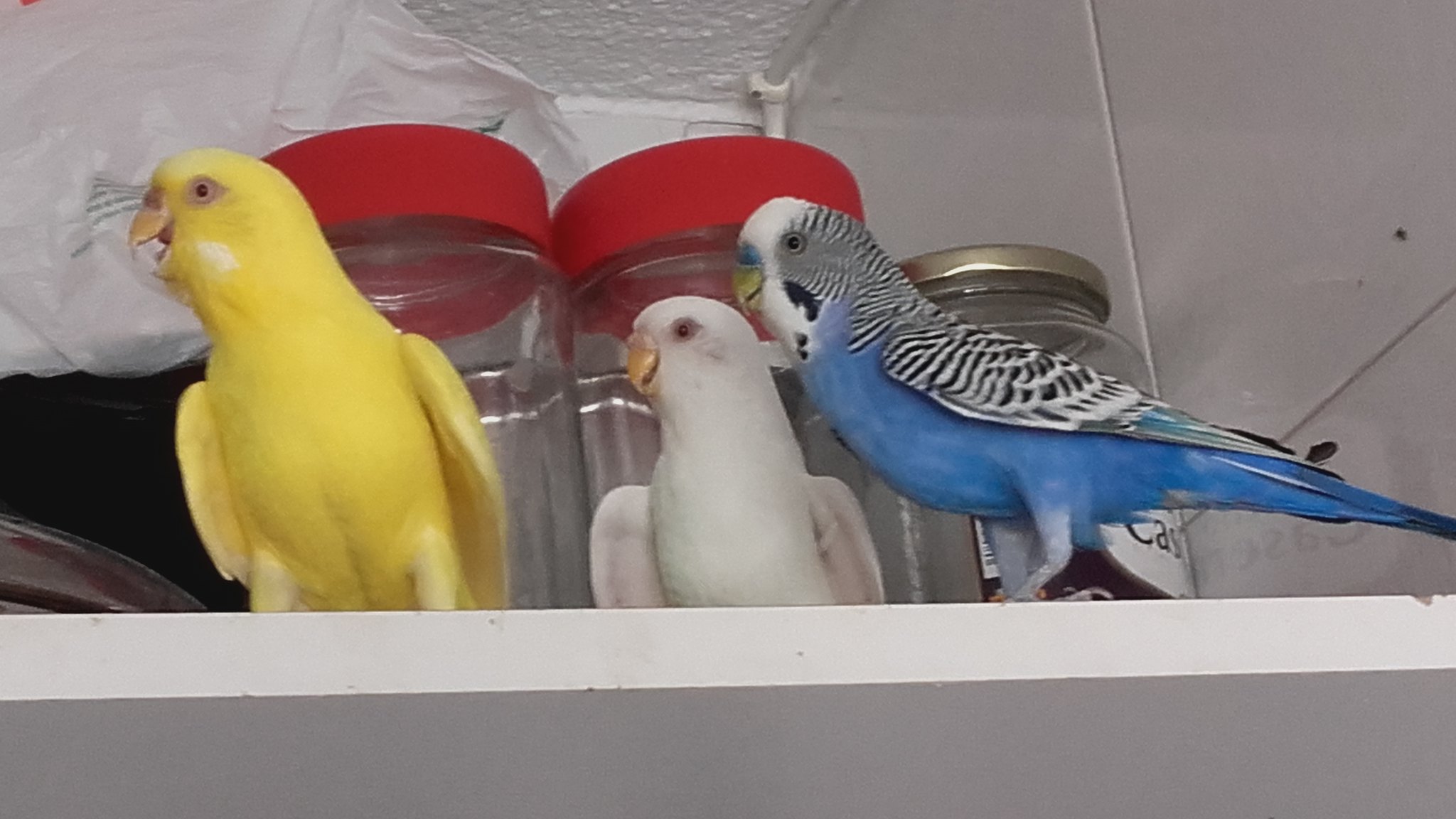This image captures three vividly colored parakeets perched on a high shelf against a backdrop of clean, white tiles and a textured white ceiling. To the upper left of the image, a plastic bag is casually placed. On the shelf behind the birds are three jars: two with red lids positioned on the left and one with a metallic lid on the right, each seemingly empty.

Focusing on the birds, the parakeet on the left is a striking yellow, with its neck extended and beak open, possibly chirping. Its small, beady eye and slightly opened wings give the impression of engagement or excitement. The middle parakeet is pure white with an orange beak, mirroring the left bird's posture by facing to the left. On the far right, the third parakeet showcases a blue body with distinctive black and white striped patterns on its wings and head. Its beak, tinged with blue and yellow, is slightly ajar. All three birds are attentively looking towards something off-camera to the left, their expressive postures suggesting curiosity or interest.